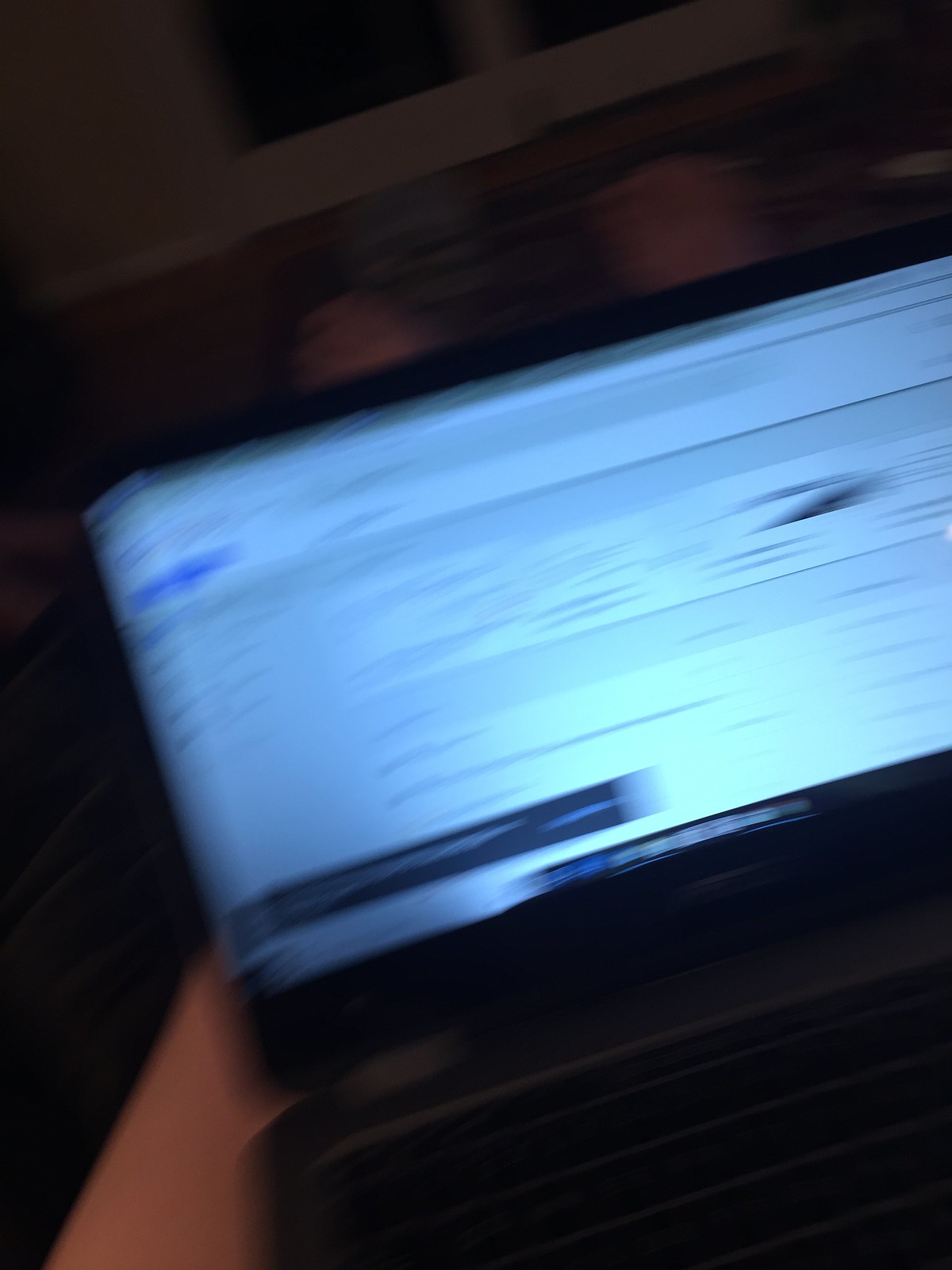The image captures a highly blurry scene of a dark gray laptop resting on someone's lap. The device is noticeably angled, approximately eight degrees to the left, showcasing its screen filled with indistinguishable text and images, possibly a Google search, bathed in digital light. The bottom part of the screen displays a prominent bar with icons, while scattered white and black squares, alongside lines of text, dominate the rest of the display. The left half of the black keyboard is visible, with the right side cropped out of the frame. The setup suggests the person is reclining, with their toes peeking up behind the screen, perhaps on a bed or a couch, illuminated by barely discernible light in an otherwise dim room. The background remains a shadowy, undefined sprawl, with hints of a wooden surface and black edges surrounding the laptop.